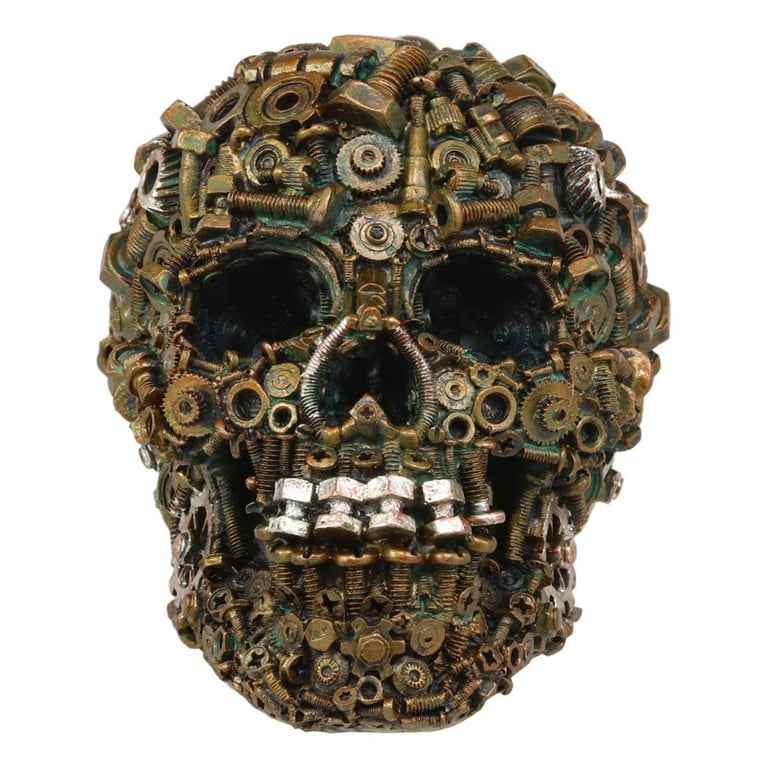This detailed image showcases a unique and intricate piece of sculpture art depicting a human skull. The artist has meticulously constructed the skull using an assortment of metal components including bolts, nuts, washers, screws, and gears. The overall color palette features a striking combination of a green patina base with copper, brass, and brownish-gold hues, accentuated by dark, hollow eye sockets that lend a deep, black appearance. The nose cavity is creatively formed using springs, while the mouth is particularly detailed, featuring upright bolts that serve as the teeth, complemented by white or silver bolts with nuts on their ends to enhance the teeth-like structure. This modern art piece creates a remarkable visual impact through its imaginative use of everyday metal objects assembled onto what appears to be a greenish background platform.